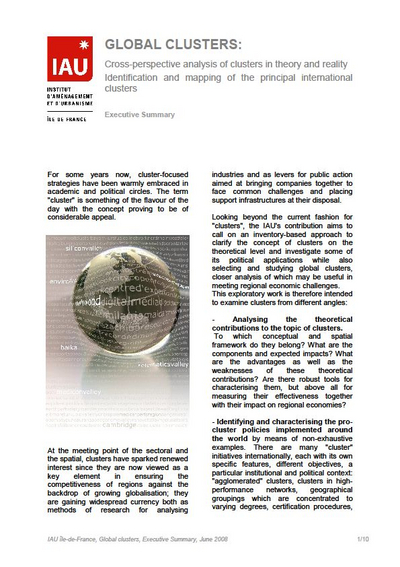### Caption for Image of Newspaper Article:

**Global Clusters Cross-Perspective Analysis: Identification and Mapping of Principal International Clusters**

In the top left corner, the logo "IAU" is prominently displayed in white against a red background, accompanied by a subtle white sun graphic. This image captures the first page of an article titled "Global Clusters Cross-Perspective Analysis of Clusters in Theory and Reality: Identification and Mapping of the Principal International Clusters." The article delves into the popular and strategic concept of clusters in academic and political realms, focusing on their importance in enhancing regional competitiveness amid growing globalization. Clusters are viewed as both research methods and public action levers for uniting companies and providing them with essential support infrastructures.

Featuring a detailed executive summary, the article traces the evolution of cluster strategies over the years. It aims to clarify the theoretical concept of clusters while investigating their political applications through an inventory-based approach. The summary highlights the need to explore clusters from various perspectives, including their theoretical foundations, components, expected impacts, and the effectiveness of these strategies on regional economies. By identifying and characterizing cluster policies across the globe, the article examines numerous cluster initiatives, each with its own objectives, institutional context, and specific features. 

The article encapsulates a comprehensive analysis, posing critical questions about clusters’ conceptual and spatial frameworks, advantages and weaknesses, and the robustness of tools used to measure their effectiveness. The executive summary concludes by promising a more in-depth exploration in the following pages, identifying this as page 1 of 10. Authored by IAU, Dider France, the article titled "Global Clusters" was published in June 2008.